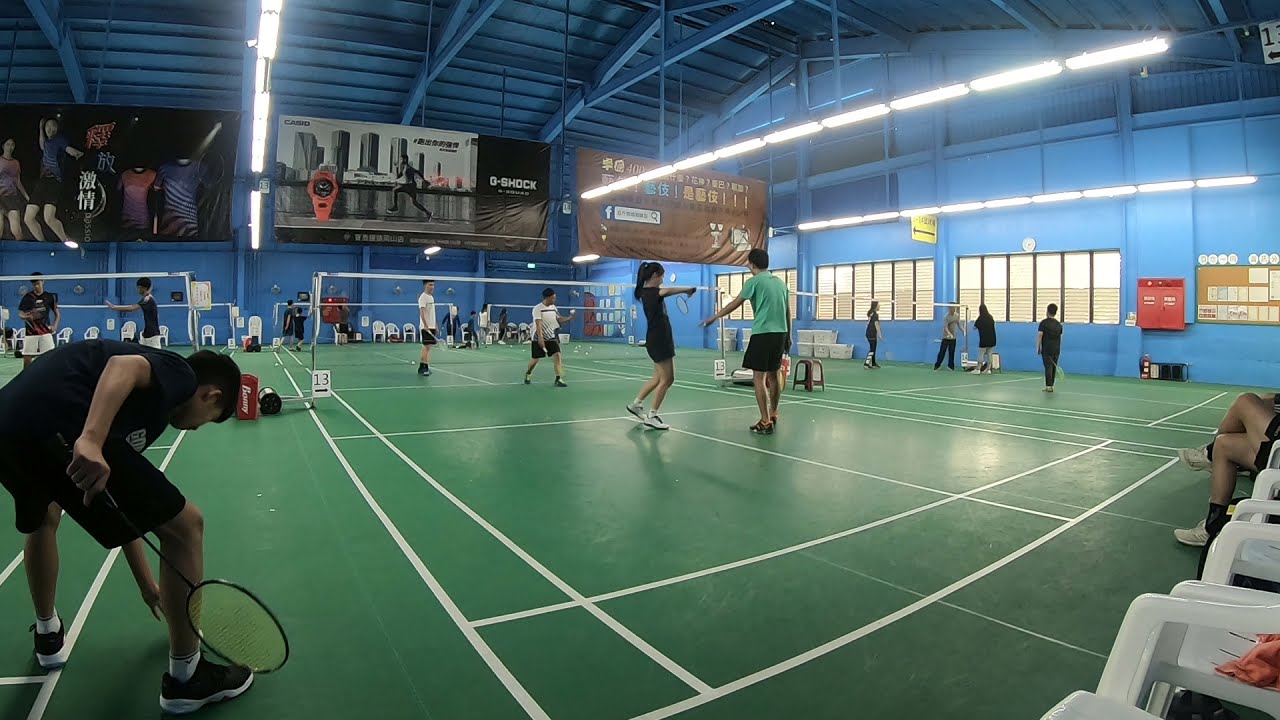In this detailed color photograph, we see the interior of a large gymnasium that is converted into a badminton arena with three distinct courts. The courts are marked by white lines on a green painted floor, and the high ceilings with visible rafters are painted blue. Along the walls, the gym features large windows and multiple hanging advertisements, including a prominent G-Shock watch ad.

In the center court, a mixed doubles game is in progress. A man and a woman on the near side of the court are playing against two men who are farther away from the viewer. Just to the left in the foreground, a young Asian man, dressed in a black t-shirt, black shorts, and black and white shoes with white socks, is bent over picking up the shuttlecock while holding his racket in his right hand.

Scattered around the gym are players either engaged in games or standing and holding their rackets, with the seating for spectators composed mainly of plastic lawn chairs positioned along the walls. The vibrant activity and details capture the essence of a bustling indoor badminton arena.